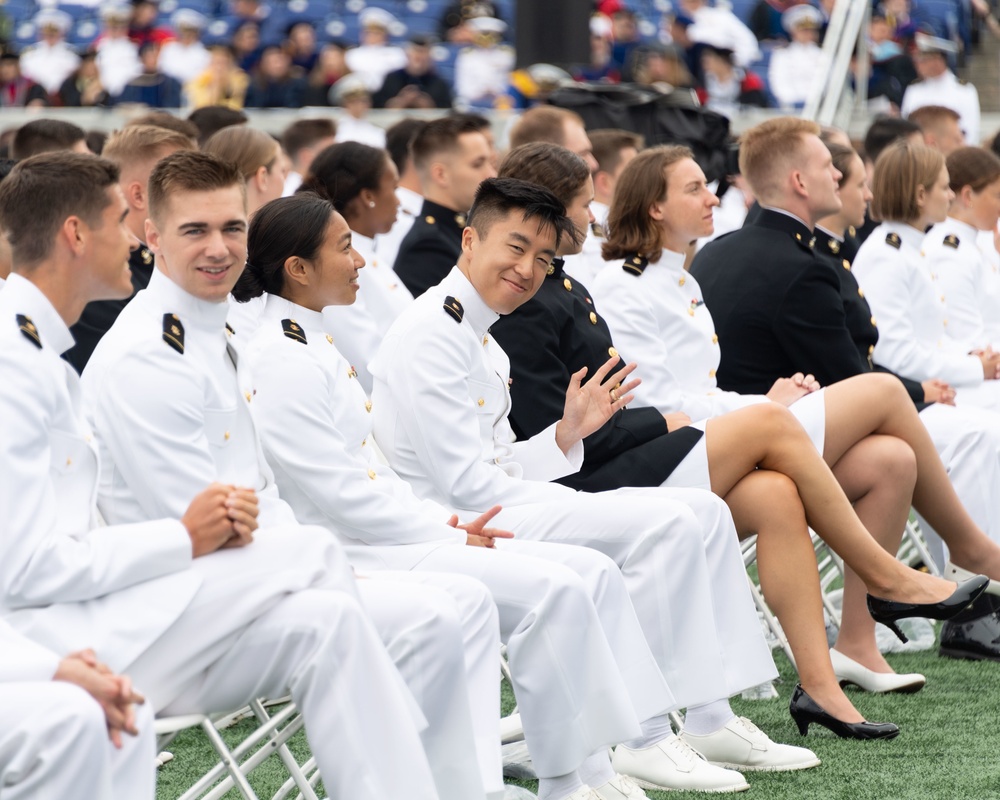The image captures a military celebration or ceremony taking place outdoors, where multiple men and women are dressed in formal military uniforms. The scene is set on a green grass turf within a stadium, with attendees seated on white chairs. The uniforms predominantly consist of white jackets with white pants, adorned with black and gold epaulettes on the shoulders. Notably, some individuals are also seen in blue uniforms with black patches. The focal point of the photograph is an Asian man in a white uniform, featuring a short cropped haircut with shaved sides and slightly longer hair on top. He is smiling warmly and waving at the camera with his left hand. In the background, spectators fill blue seats in the stadium stands, observing the event.